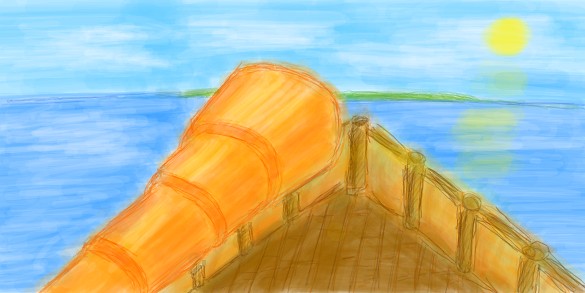This crayon drawing features a serene coastal scene. The background showcases a blue sky with a radiant yellow sun shining from the right. Below, the ocean glistens in a vibrant blue, extending to a sliver of green land visible on the horizon. The primary focus of the piece is the bow of a wooden boat, crafted with detailed brown beams and wooden slat flooring. Prominently mounted on the bow is a large, golden telescope, directed towards the distant island and sun, suggesting a sense of adventure and exploration.